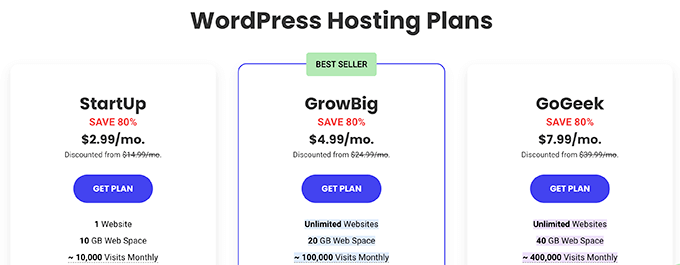This is a screenshot of a website showcasing WordPress hosting plans, prominently presented with bold black text at the top. The three subscription options are displayed in three distinct columns below the heading.

- **Left Column - StartUp Plan:**
  - **Promotion:** Save 80%
  - **Price:** $2.99/month, discounted from $14.99/month
  - **Button:** "Get Plan" in a purple box
  - **Features:** 
    - Suitable for one website
    - Provides 10 GB of web space
    - Supports 10,000 visits per month

- **Middle Column - GrowBig Plan:**
  - **Label:** Bestseller (indicated with bold text and outlined in purple)
  - **Promotion:** Save 80%
  - **Price:** $4.99/month, discounted from $24.99/month
  - **Button:** "Get Plan" in a purple box
  - **Features:**
    - Supports unlimited websites
    - Offers 20 GB of web space
    - Supports 100,000 visits per month

- **Right Column - GoGeek Plan:**
  - **Promotion:** Save 80%
  - **Price:** $7.99/month, discounted from $39.99/month
  - **Button:** "Get Plan" in a purple box
  - **Features:**
    - Supports unlimited websites
    - Provides 40 GB of web space
    - Supports 400,000 visits per month

Note: Each column appears to be truncated, indicating that this screenshot does not capture the complete content of the webpage. A small white box surrounds each column, but the edges are visibly cut off.